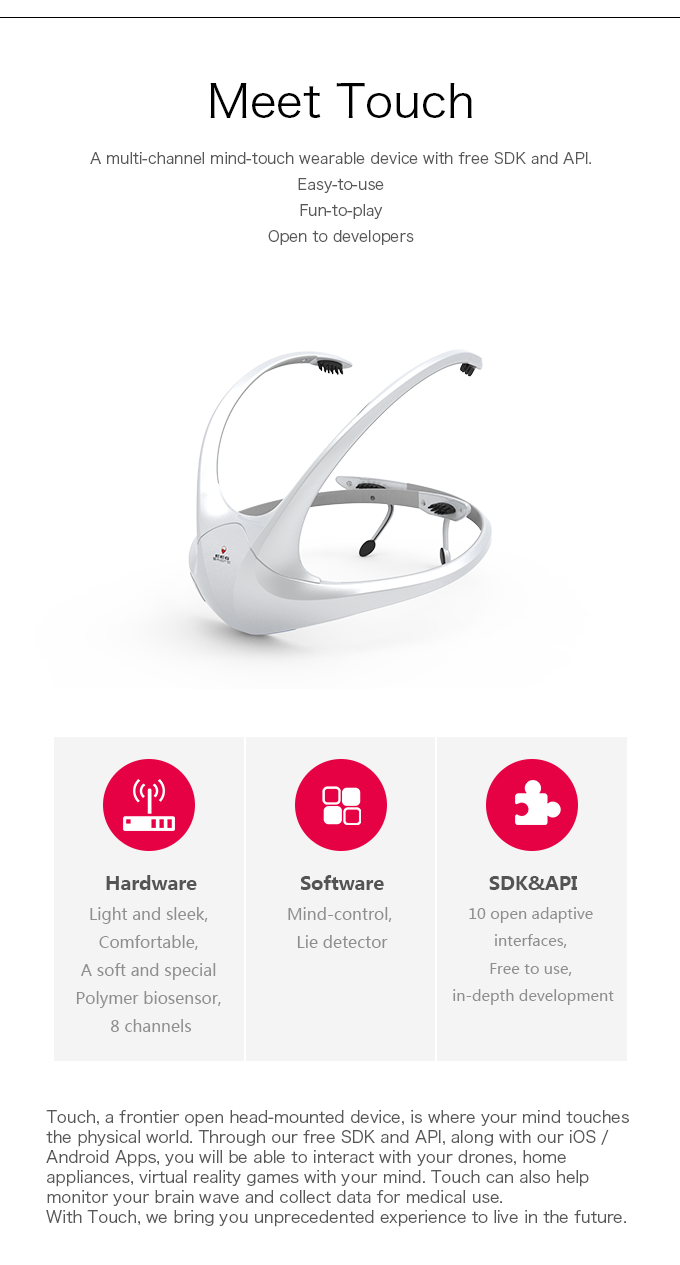Here is a polished and detailed caption based on the provided description:

---

Screenshot of the MeetTouch Device: 

The image features a multi-channel, mind-touch wearable device named MeetTouch, which is designed for ease of use and development flexibility. The MeetTouch device is predominantly white with two antenna-like structures extending from the top and a circular halo towards the bottom. There are black elements where the device connects to the head, likely for both comfort and stability.

Below the image of the device, the screenshot showcases three informative sections:

1. **Hardware**: Encased in a light gray box, this section highlights the device's sleek and comfortable design, featuring a special polymer biosensor. The hardware includes an icon of a square with an antenna emitting signals, emphasizing its capabilities. Key points mentioned are "light and sleek," "comfortable," "soft and special polymer biosensor," and "eight channels."

2. **Software**: This section is marked by a red circle containing four small squares, where two are fully shaded and the other two are outlined, displayed diagonally from each other. It focuses on the software capabilities of the device, noting "mind control" and "light detector."

3. **SDK and API**: Represented by an icon of a puzzle piece within a red circle, this section underscores the development potential of the device with "10 open adaptive interfaces," "free to use," and "in-depth development."

The page layout is simple, featuring a white background with a paragraph at the bottom, adding to the clean and minimalistic design.

---

This caption provides a comprehensive and structured overview of the device, highlighting its design, functionality, and development features.